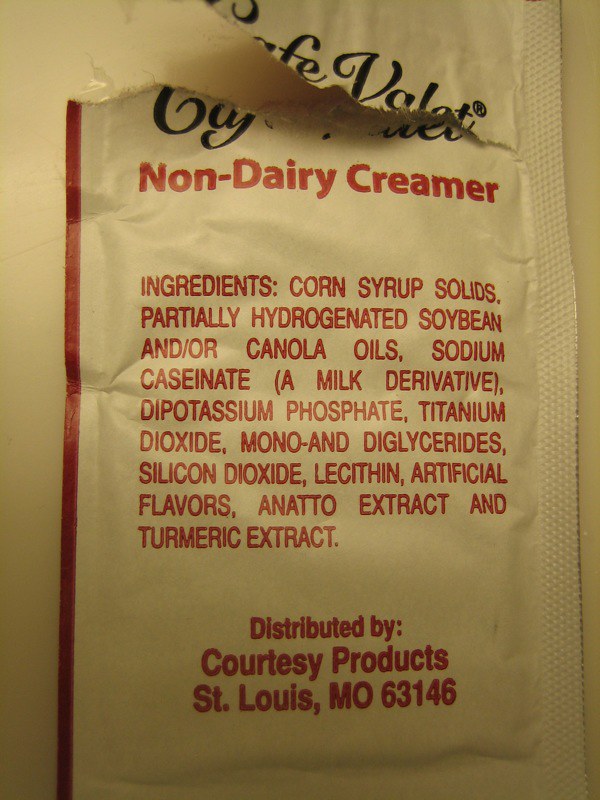This image showcases a torn, single-serving packet of non-dairy creamer from the brand Cafe Valet. The packet is primarily white with a maroon red trim on the left side. At the top, the brand name "Cafe Valet" is displayed in an elegant black script font. Below it, "non-dairy creamer" is printed in red. The ingredients, also listed in red, include: corn syrup solids, partially hydrogenated soybean and/or canola oils, sodium caseinate (a milk derivative), potassium phosphate, titanium dioxide, mono and diglycerides, silicon dioxide, lecithin, artificial flavors, annatto extract, and turmeric extract. Additional text at the bottom states that the product is distributed by Courtesy Products, based in St. Louis, Missouri, zip code 63146.